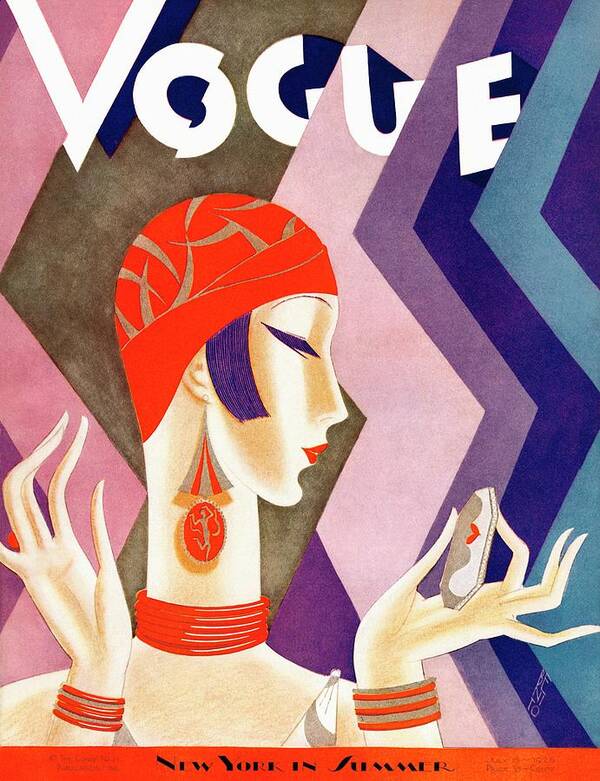This intricate image portrays a vintage Vogue magazine cover, likely from the mid-1900s. A chic woman, highly stylized in a chalk drawing manner, graces the center. Her profile features a poised expression with eyes closed, looking down to the right. She dons a tight-fitting red turban-style cap embellished with elaborate gold designs, from which a hint of purple hair peeks out.

Her neck is adorned with a striking multi-ringed red choker that complements the red bangles on her spindly wrists. She is depicted holding a compact mirror, delicately pinched between her long fingers. Her elongated neck and extravagant jewelry, including silver and red tasseled earrings with a pendant figure, emphasize her elegance. 

The vibrant background is alive with geometric zigzag patterns in hues of salmon pink, tan, violet, muted purple, and various shades of blue, enhancing the central figure's prominence. At the top of the cover, the word “Vogue” is emblazoned in bold white letters, while the bottom features a red banner with the text "New York in Summer." A discrete signature, seemingly "Benito," completes this high-fashion artwork.